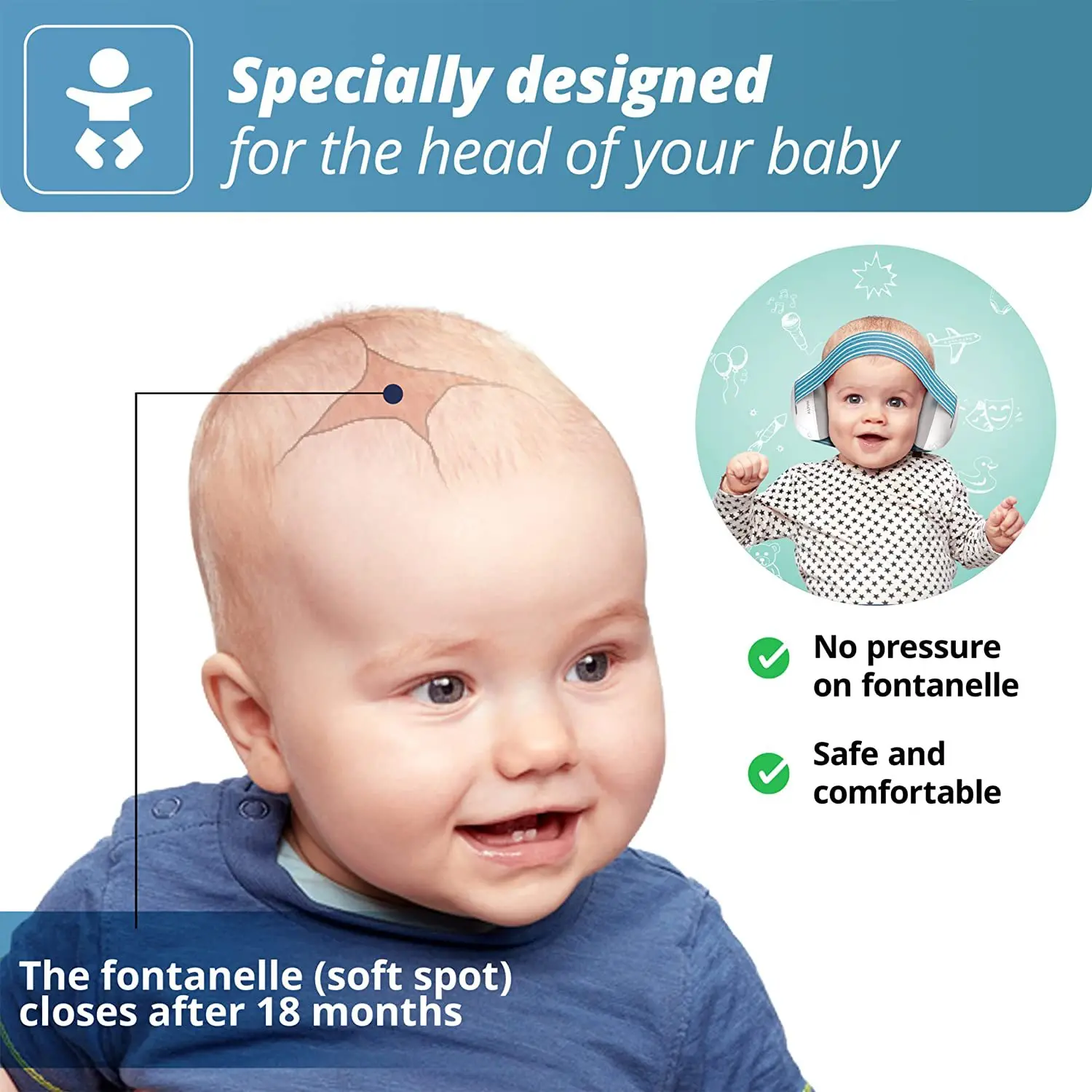This is a detailed advertisement for baby headphones designed to protect the soft spot on a baby's head. Along the top of the ad, a blue banner displays in white text: “Specially designed for the head of your baby,” accompanied by a baby icon. Central to the composition is an image of a smiling baby with blue eyes, wearing a blue t-shirt with a lighter blue one underneath. The baby has two bottom teeth and is marked with a line indicating the fontanelle, or soft spot, which closes after 18 months.

To the right, an inset circular image showcases the baby wearing the headphones, which are white with gray padding and feature a blue strap running along the forehead rather than over the top of the head. The headphone design emphasizes that there is “No pressure on the Fontanelle,” ensuring they are “Safe and comfortable” for the child. The ad includes line art in the background featuring playful elements like balloons, a microphone, a sun, an airplane, and masks, enhancing the cheerful and considerate design of the product.